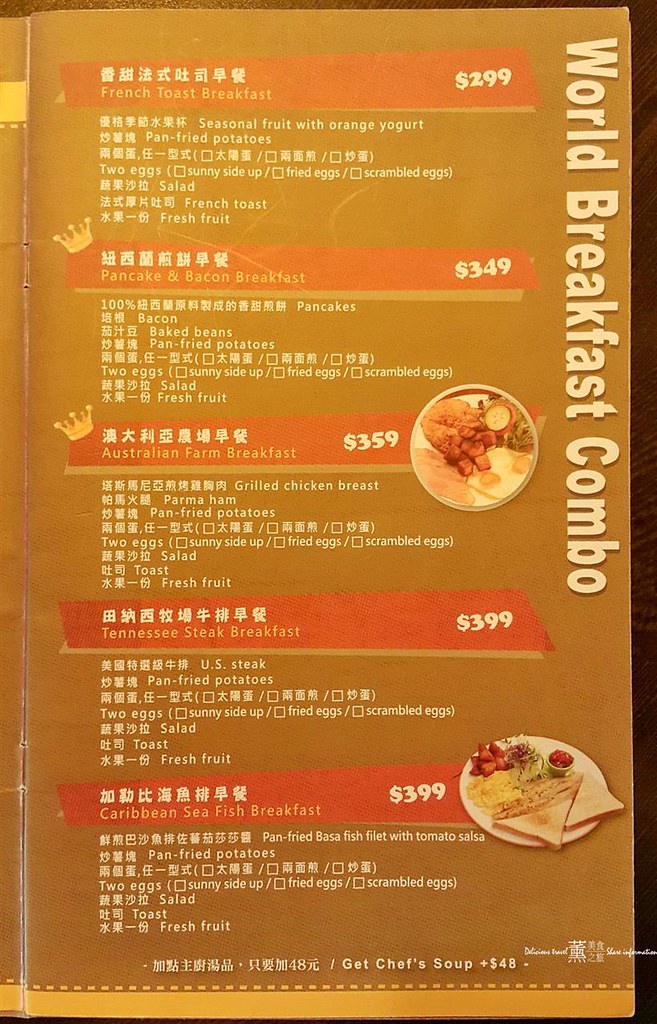The image showcases a menu with both Asian language script and English text, set against a brown backdrop with various orange banners detailing different breakfast options. Down the right margin, "World Breakfast Combo" is printed in light yellow.

1. At the top of the menu, the first orange banner reads "French Toast Breakfast" with Asian characters above it, priced at $2.99. The listed items include:
   - French Toast
   - Seasonal Fruit with Orange Yogurt
   - Pan Fried Potatoes
   - Two Eggs Sunny Side Up
   - Fried Eggs
   - Scrambled Eggs
   - Salad
   - Fresh Fruit

2. Below it, another orange banner is crowned with a crown symbol and states "Pancakes and Bacon Breakfast" for $3.49. The menu items below, indicated in both English and Asian language, consist of:
   - Pancakes
   - Bacon
   - Baked Beans
   - Pan Fried Potatoes
   - Two Eggs Sunny Side Up
   - Fried Eggs
   - Scrambled Eggs
   - Salad
   - Fresh Fruit

3. The next section features an orange banner with a crown symbol in the upper right corner. It advertises the "Australian Farm Breakfast" for $3.59, accompanied by a circular image of food. Below, the listed items are:
   - Grilled Chicken Breasts
   - Parma Ham
   - Pan Fried Potatoes
   - Two Eggs Sunny Side Up
   - Fried Eggs
   - Scrambled Eggs
   - Salad
   - French Toast
   - Fresh Fruit

4. Following that, an orange stripe details the "Tennessee Steak Breakfast" at $3.99. The items available are:
   - U.S. Steak
   - Pan Fried Potatoes
   - Two Eggs Sunny Side Up
   - Fried Eggs
   - Scrambled Eggs
   - Salad
   - French Toast
   - Fresh Fruit

5. At the bottom, the "Caribbean Seafish Breakfast" is displayed with an image of a plate containing toast, eggs, and fruit. It is described with:
   - Pan Fried Basa Fish with Tomato Salsa
   - Pan Fried Potatoes
   - Two Eggs Sunny Side Up
   - Fried Eggs
   - Scrambled Eggs
   - Salad
   - Toast
   - Fresh Fruit

Additionally, it is mentioned that for an extra $0.48, one can get "Chef Soup."